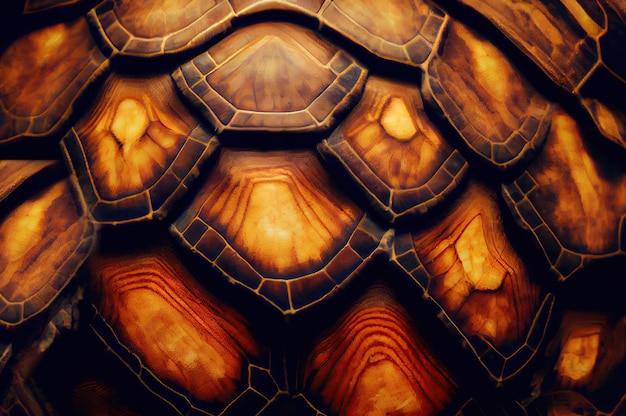The photograph captures a highly detailed and close-up view of an intricate piece of artwork reminiscent of a turtle shell, constructed from finely carved and burnt wood. The image showcases interlocking hexagonal and polygonal shapes, arranged to mimic the scaled pattern of a turtle's back. The wooden pieces are polished to a high sheen, exhibiting a gradient of colors: light brown centers with dark brown and almost blackish-brown outer edges, separated by thin white lines that create distinct borders around each shape. The shapes appear to be trapezoidal with curved bottoms, layered one over the other in a shingle-like manner, contributing to a slightly domed appearance with a higher middle. The rich coloration melds amber, browns, golds, and dark yellows, set against a predominantly black background, enhancing the artwork's ornate and decorative appeal. The bottom left and right corners of the image are particularly dark, emphasizing the intricate details of the central design.